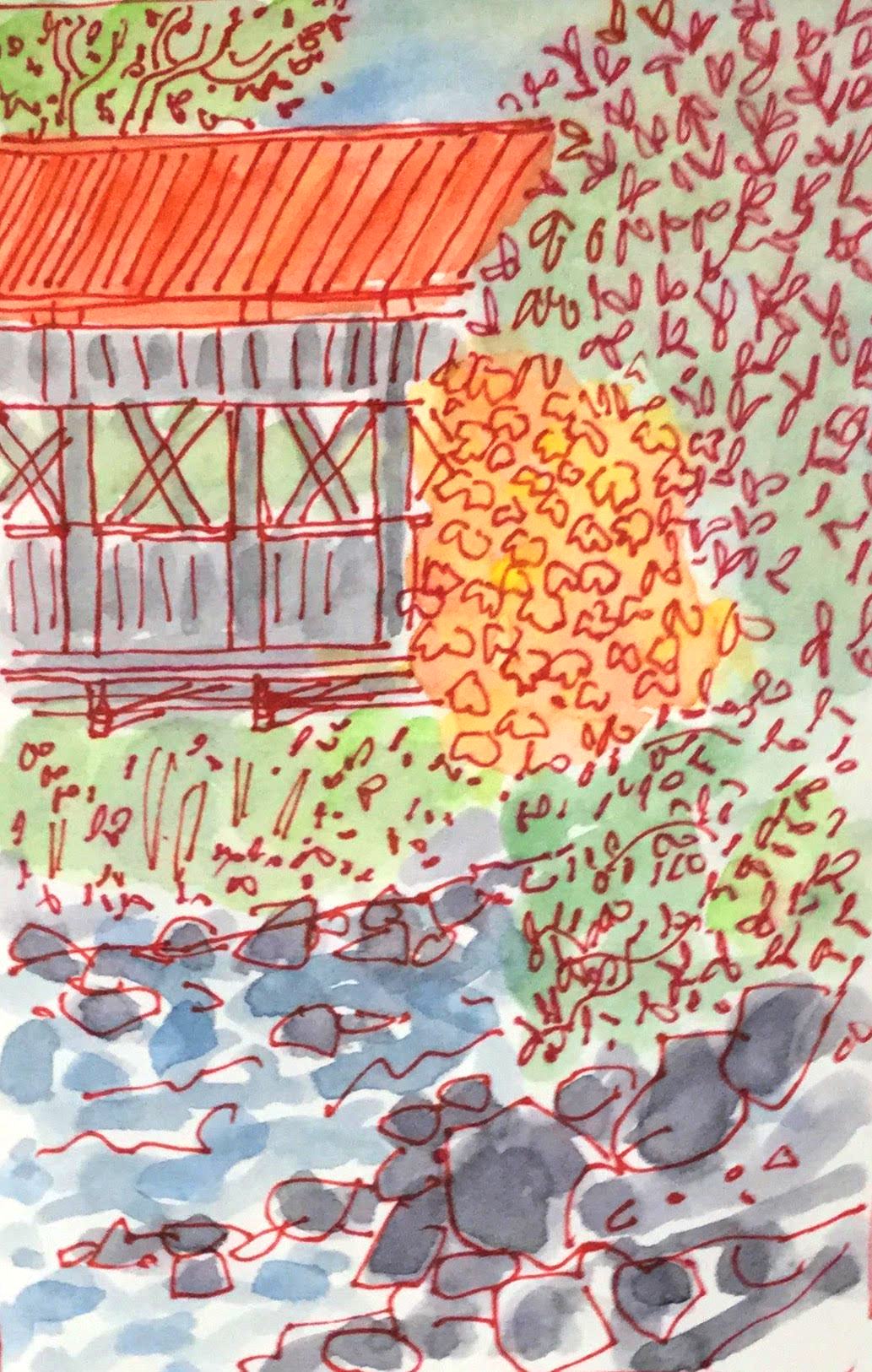This is a detailed watercolor painting accentuated with brown pencil drawings, depicting a serene autumn scene centered around a charming covered bridge. The bridge is nestled among trees, whose branches, trunks, and leaves are intricately drawn with brown pencil squiggles to symbolize foliage, and are enveloped in vibrant green and yellow watercolors. The foreground features a stream, portrayed with light blue watercolor to signify water, interspersed with gray spots that signify rocks, outlined with brown pencil for added texture.

The covered bridge itself boasts a red-orange roof, illustrated with brown pencil lines to represent wooden slats, whereas the underside is rendered in gray watercolor with brown lines indicating metal slats. Each window formation of the bridge is detailed with an X-shaped design, reinforced by a gray metal fence up to the midpoint with brown lines, likely signifying wooden slats. The bridge trusses underneath add structural realism to the depiction.

Surrounding one side of the bridge is a lawn, highlighted with brown squiggles suggestive of fallen leaves, enhancing the seasonal ambiance of the artwork. The intricate blend of watercolor and brown pencil drawings brings a rich, textured quality to this tranquil fall landscape.